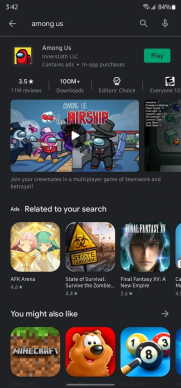The image appears to be a blurry screenshot taken from an Android device at the time of 3:42, although it's not clear if it's AM or PM. The top portion of the screen displays a battery status indicating 84% charged. Below this, an arrow pointing left signifies navigating back, with "Among Us" typed into a search bar that includes a white magnifying glass icon and a microphone icon. 

Underneath the search bar, there's a yellow square icon featuring a red mask, adjacent to a label that reads "Among Us" in white text, followed by "Contains ads · In-app purchases." Below this, a green rectangular button with "Play" written in black, indicates the option to start the game. The game has a rating of 3.5 stars with 11 million reviews and over 100 million downloads. It's labeled as "Editor's Choice" and rated for "Everyone."

Further down, there is a video preview indicated by a white play button overlaid with "Airship" in red text. Several "Among Us" characters are displayed, including a pink character, a silver one, and a gray one with a hat. Below this, the section "Related to your search" includes game titles such as "Final Fantasy: State of..." (partially visible), "AFK..." (partially visible), and "Minecraft" listed at the bottom under "You might also like." The incomplete text suggests partial visibility of these recommendations.